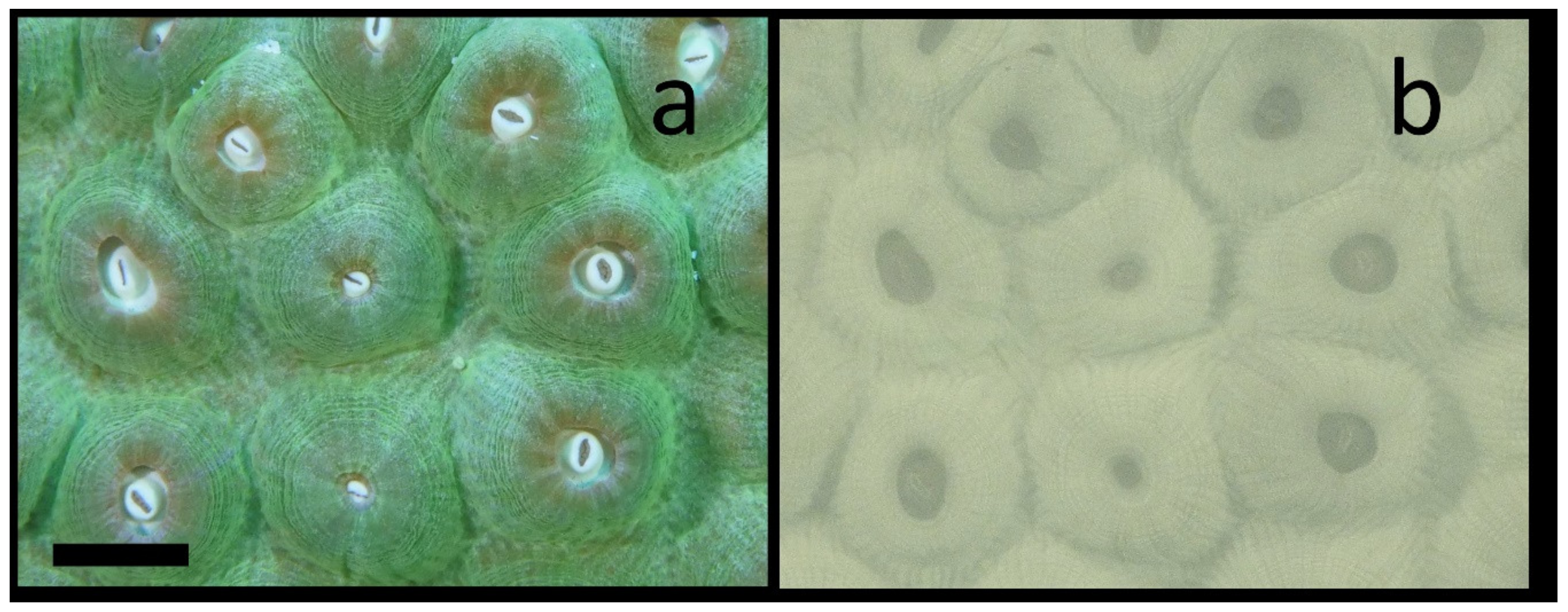This is a side-by-side image set, possibly depicting specimens under magnification or a microscope. The images are labeled A and B, with each occupying one half of a rectangular frame, split by a vertical black line. Image A, on the left, exhibits vibrant shades of green, featuring about eight rounded, blobby structures clustered together, possibly resembling barnacles, coral polyps, or anemones. Each rounded section has a white or beige central part, akin to a mouth or suction cup, creating a texture comparable to the exterior of a pineapple without its spines. Notably, this image has a black bar at the bottom, possibly obscuring some text or a label. Image B, on the right, mirrors the arrangement of Image A but appears as a highly blurred and desaturated version, showcasing similar shapes in washed-out beige and white tones, akin to a negative image of the left. This set might be used for educational purposes, promoting a comparison of the same biological structures under different conditions or filters.